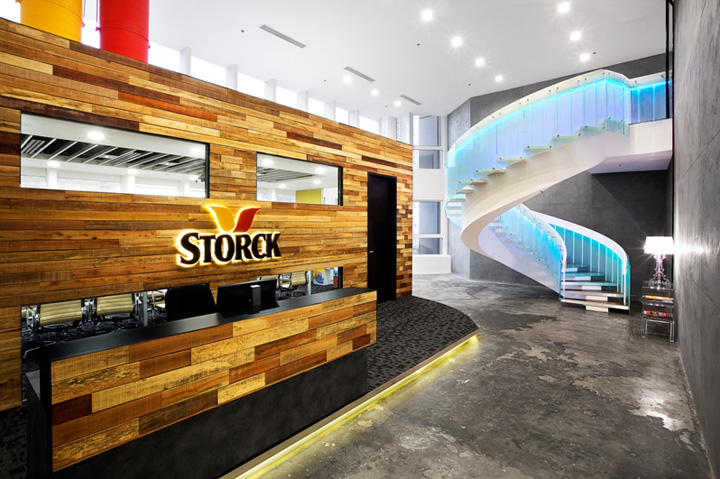This photograph showcases the interior of a modern office building or store, featuring prominently in the center a striking wooden wall composed of multi-colored panels. On this wall, the word "STORCK" is displayed in bold black letters, accented with a distinctive red and yellow design above the 'O' and 'R'. Directly beneath this sign is a long black desk equipped with a computer and chair, all positioned on top of a sleek black platform illuminated by gold lights underneath. The flooring throughout the space is a refined gray marble, and to the right, there's a concrete wall. A unique spiral staircase with white steps and neon bluish-green illumination, adorned with holographic blue rails and white handrails, adds architectural interest. Adding a touch of coziness, a small table with a lamp is placed down below the staircase. White ceilings and a white back wall complete the contemporary and polished aesthetic.